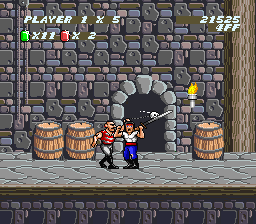The image captures a screenshot from a classic video game, reminiscent of titles from the 1980s or 1990s. The setting appears to be within a medieval dungeon or castle, characterized by its rugged stone walls. Three meticulously detailed brown barrels, complete with wooden grain lines, are placed against the backdrop. A torch with a vivid orange flame is mounted next to an arched doorway, which is framed by sturdy stone blocks. Two cartoonish male characters are positioned near the doorway, seemingly engaged in combat. In the screen's upper left corner, a HUD element displays "Player 1, X5," suggesting the player's lives or attempts remaining. Below this, a green gemstone icon marked "X11" and a red gemstone with "X2" hint at collectible items or power-ups. Additional numerical information is visible in the upper right corner, though its purpose remains unclear, likely related to scoring or game statistics.